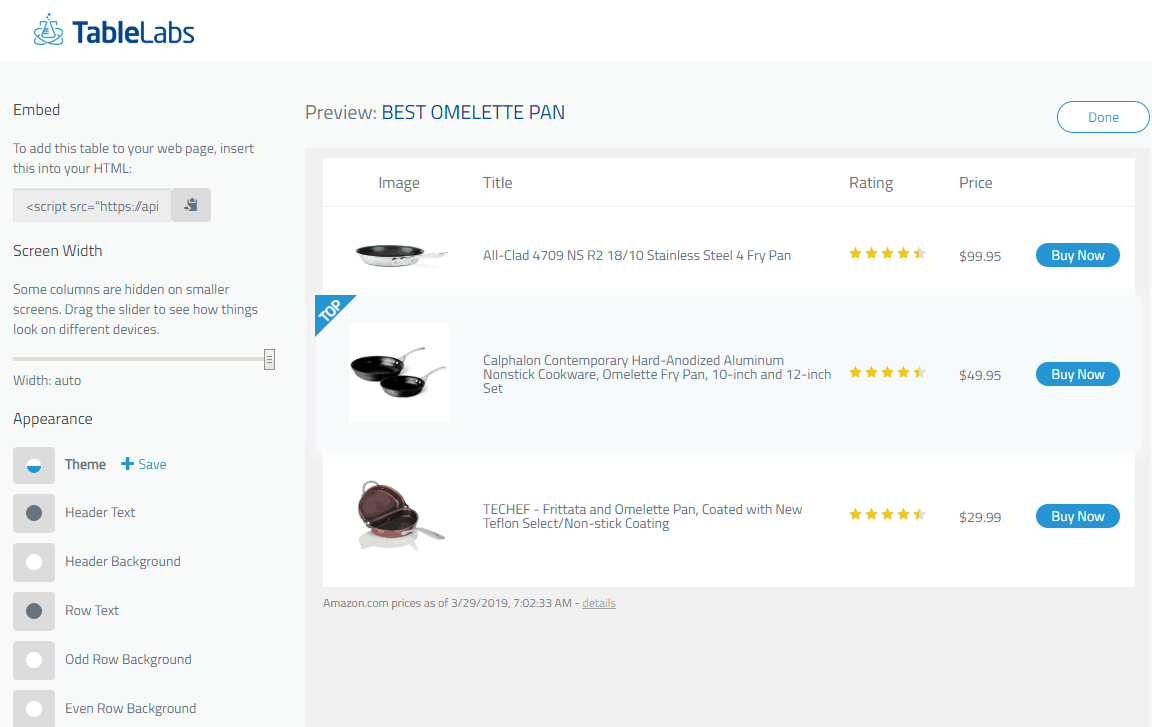This image is a detailed screenshot from TableLabs showcasing a comparison table titled "Preview Best Omelette Pan." In the top left corner, the TableLabs logo is prominently displayed. The table is organized into columns that feature an image, title, rating, and price for each product. 

1. **All-Clad 4709NSR218-10 Stainless Steel Fry Pan**: 
   - **Image**: Stainless steel frying pan.
   - **Rating**: 4.5 stars, displayed with yellow stars.
   - **Price**: $99.95.
   - **Additional Feature**: Blue "Buy Now" button.

2. **Calphalon Contemporary Hard-Anodized Aluminum Non-Stick Cookware Omelette Fry Pan (10 and 12 inch set)**: 
   - **Image**: Two non-stick fry pans.
   - **Rating**: 4.5 stars.
   - **Price**: $49.95.
   - **Additional Feature**: Blue "Buy Now" button.

3. **Tech Chef Fridia and Omelette Pan Coated with New Teflon Select/Non-Stick Coating**: 
   - **Image**: Non-stick omelette pan with a folding feature.
   - **Rating**: 4.5 stars.
   - **Price**: $29.99.
   - **Additional Feature**: Blue "Buy Now" button.

To the left of the table, there are instructions for embedding the table on your own website, as well as a screen width slider for resizing the table. The prices shown are noted to be from Amazon.com, accurate as of March 29, 2019, at 7:02:33 AM.